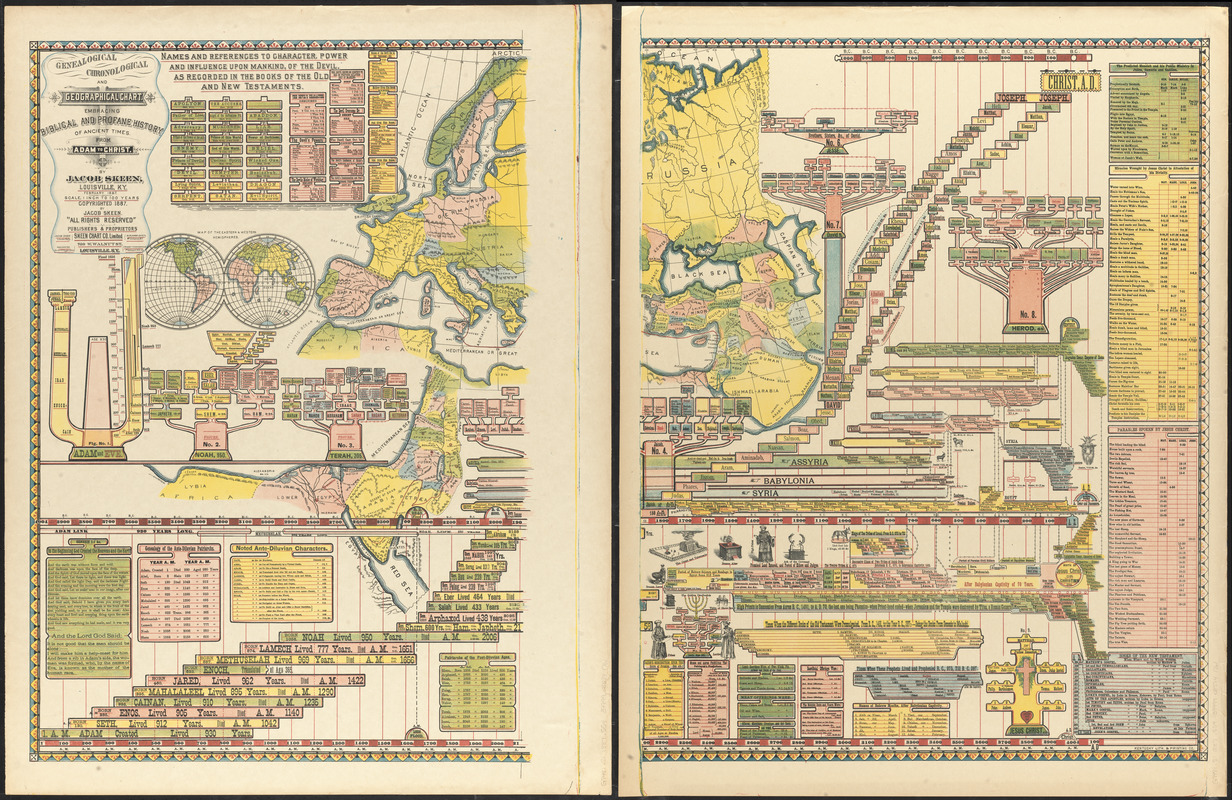This detailed image features a vintage-style map with a pale peach background, divided into two main sections separated by a black line. It displays both circular and flat depictions of global maps, framed with intricate brackets of information in pink, green, and yellow shades. The upper left corner of the image reads "Genealogical, Chronological, and Geographical Chart: Biblical and Profane History of Ancient Times," attributed to Jacob Skeen of Louisville, Kentucky, with all rights reserved. The map is adorned with numerous charts and timeline graphs illustrating biblical and profane history from Adam to Christ. In the top section, text discusses names and references to the character, power, and influence of the devil as recorded in the Old and New Testaments. The image is densely packed with visuals and text, making it hard to discern smaller details and fonts.